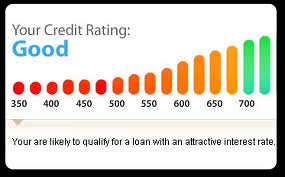The image is a small, colored advertisement with a white background and black border, depicting a detailed graph of credit ratings. The title "Your Credit Rating" appears at the top, with the word "Good" highlighted in blue below it. The graph consists of bars that grow in size corresponding to credit scores ranging from 350 to 700, with the colors transitioning from red at the lower end, through orange and yellow, to green at the higher end. The x-axis of the graph is marked with increments of 350, 400, 450, 500, 550, 600, 650, and 700. Below the graph, the text reads "You are likely to qualify for a loan with an attractive interest rate." Despite being a bit pixelated and blurry, the graphic clearly aims to convey the significance of one's credit score in loan qualification.